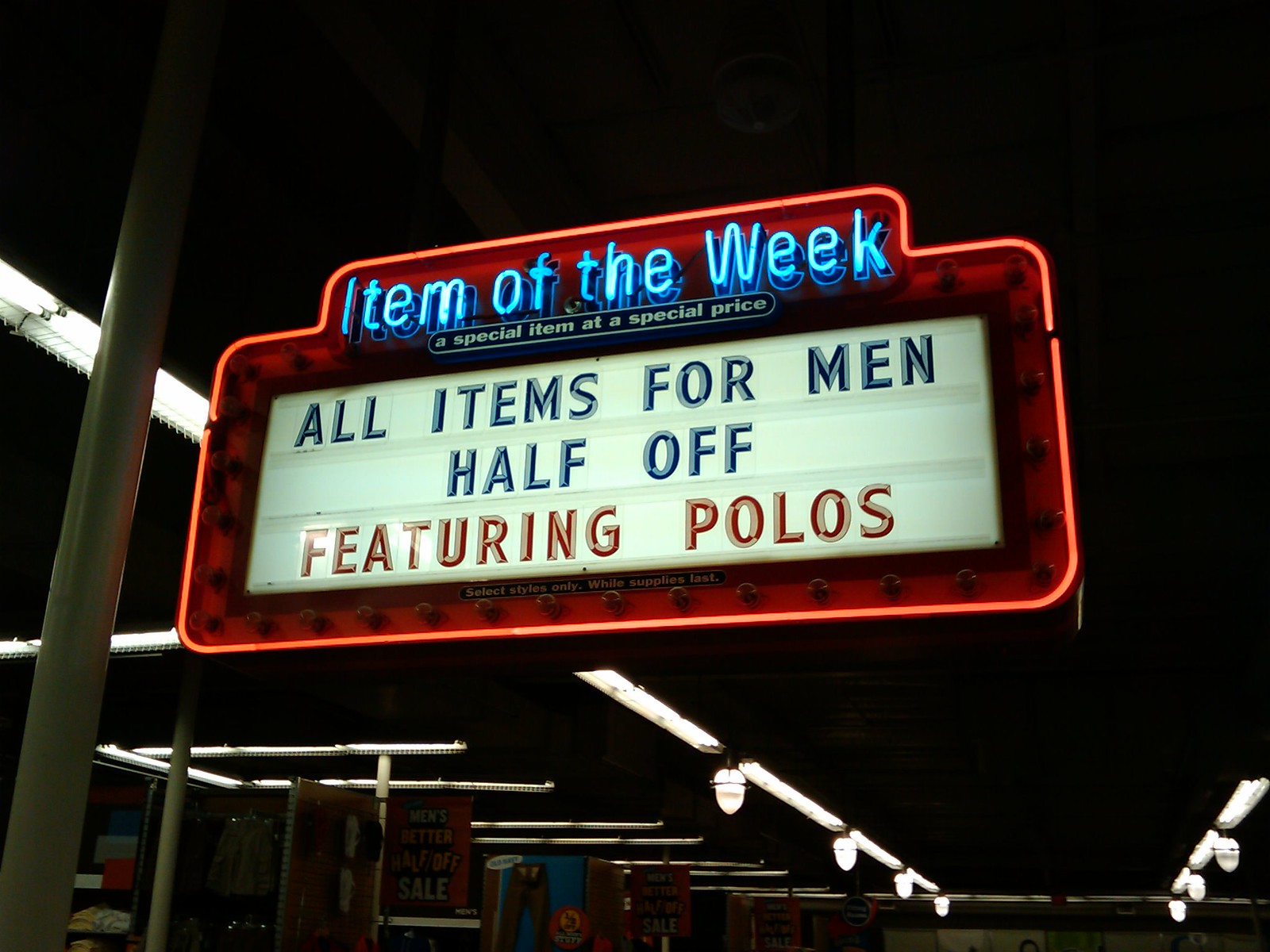This is a photograph taken at night of a neon marquee sign, likely in a shopping area or retail outlet. The background is predominantly dark, illuminated by various fluorescent lights and sporadically placed lanterns. The sign is designed to evoke the feel of an old diner or movie theater marquee, featuring a vibrant red neon border that gives it a distinctive glow. Across the top of the sign, in bright blue neon, it reads: "ITEM OF THE WEEK." Below this, in non-lit text, it says: "A SPECIAL ITEM AT A SPECIAL PRICE." Continuing down, on a retro-style flat white background, blue uppercase lettering announces: "ALL ITEMS FOR MEN HALF OFF." Below that, in red uppercase lettering, it declares: "FEATURING POLOS." The sign itself appears to be mounted on a pole to the left side, with other poles and white lights visible in the distance, enhancing the sense of a bustling retail environment.